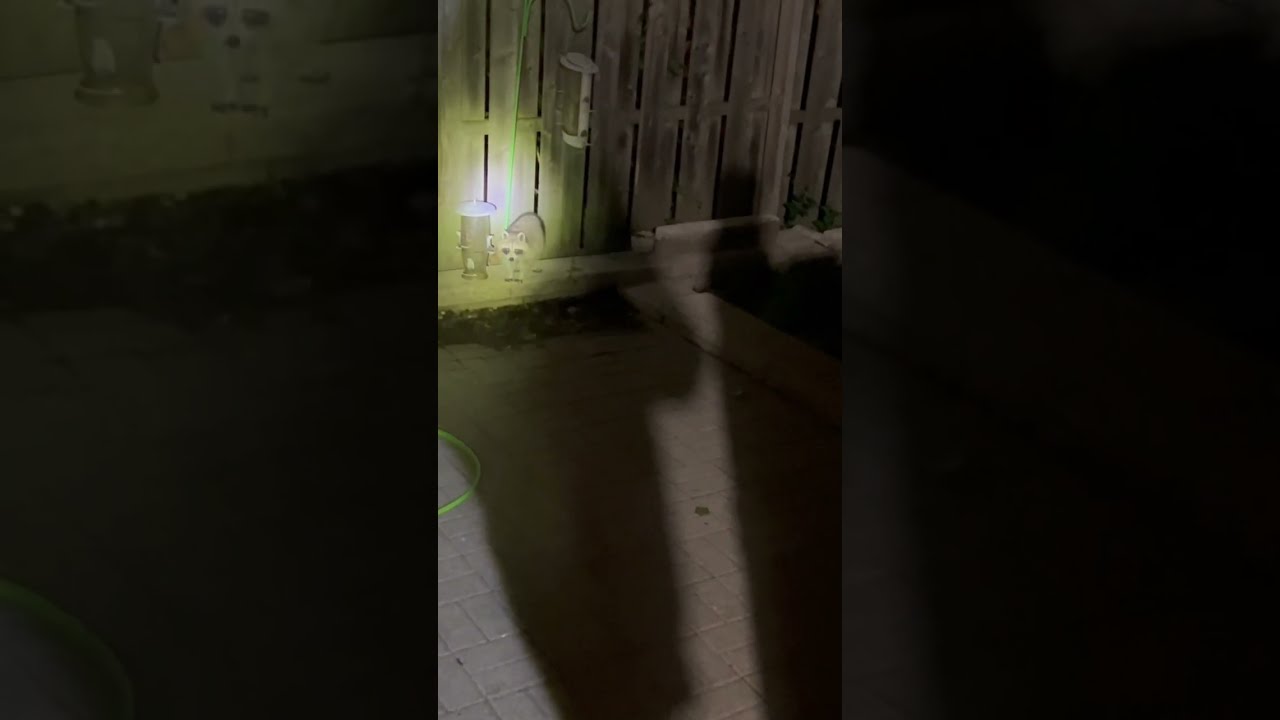The image features a nighttime scene, depicted in a triptych of vertically oriented rectangular photos. The central panel presents the complete picture: a backyard with a tan wooden fence in the background, subtly illuminated by a nearby light source. Shadows, likely of the photographers, stretch across a brick patio that extends into a small garden area at the edges. Front and center, in the direct light, stands a raccoon, next to a metal hook presumably used for a bird feeder.

The left and right panels provide zoomed-in views of the corresponding sections of the central image, though they appear darker with less lighting. The left panel continues the brick patio and hints at what might be a garden figurine, while the right panel focuses on the raccoon against the fence background. This triptych, captured vertically, accentuates the details of a calm backyard scene under soft night lighting.